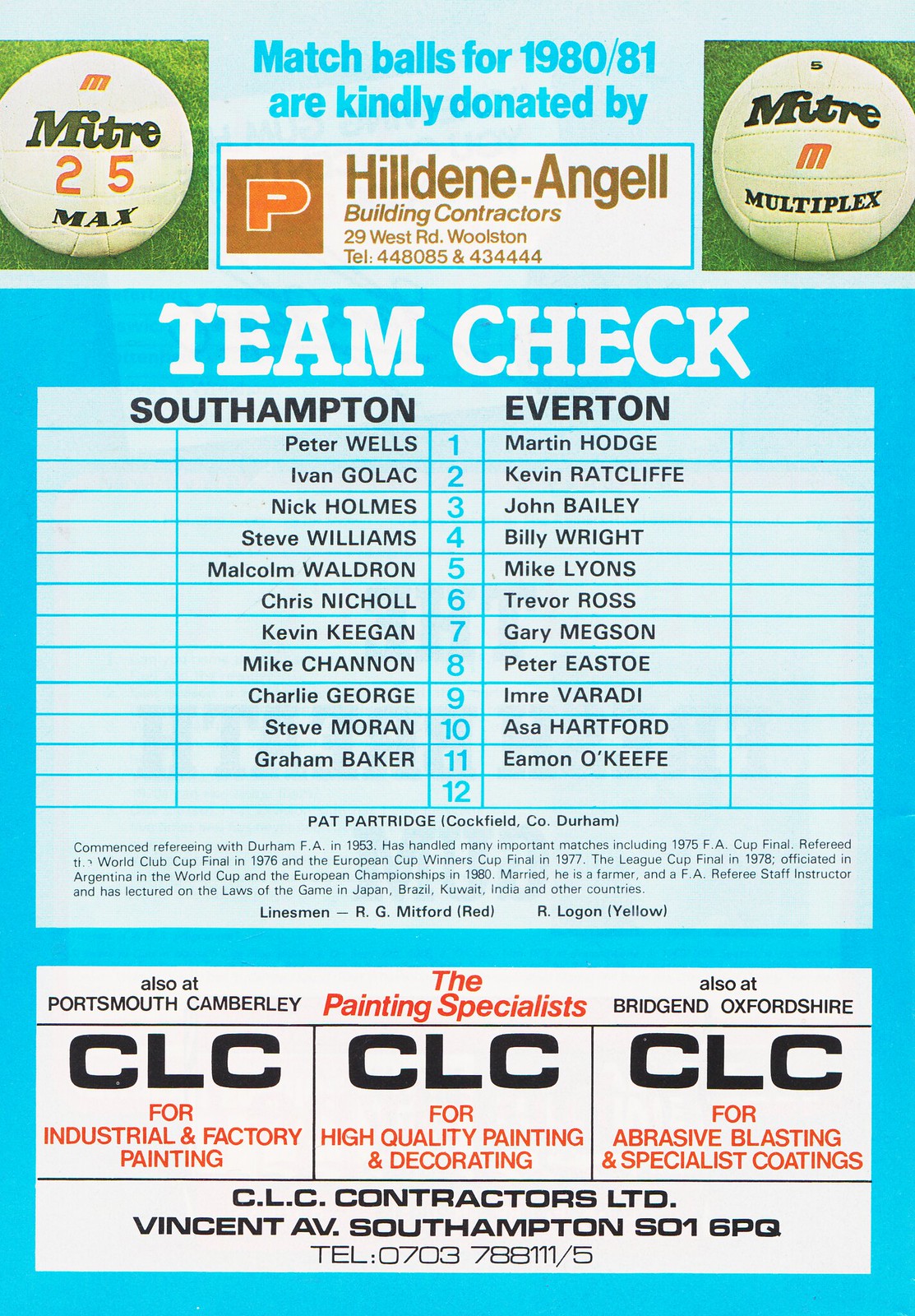This full-color image is from a soccer program featuring details about a sporting event. In the upper left and right corners, there are pictures of soccer balls, one labeled "MITRE 25 Max" and the other "MITRE M Multiplex." Central to the top section, in darker blue lettering on a light blue background, is the text: "Match balls for 1980-81 are kindly donated by Hildene Engel Building Contractors." Just below this, on a bright blue background with white lettering, is a label that reads "Team Check." Below this label, the page is divided into two columns: the left column lists the names and numbers of Southampton players, while the right column is intended for Everton players but contains no names or numbers. The bottom of the image includes advertisements for various services, such as "Plymouth Chamberley," "CLC Contractors Limited for industrial and factory painting, high-quality painting and decorating, abrasive blasting and specialist coatings," and also provides the address and contact information for CLC Contractors Limited at Vincent Ave, Southampton SO1 6PQ.